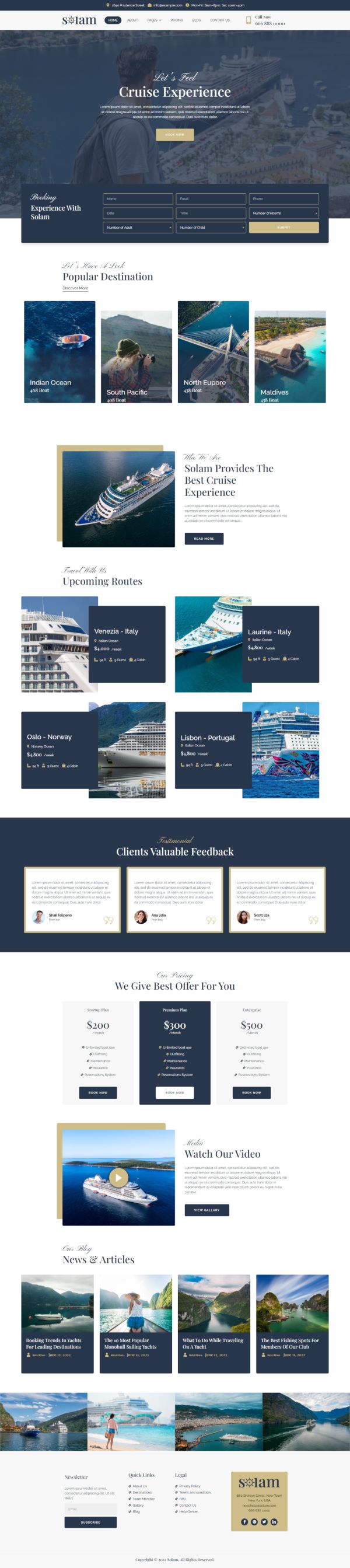This image depicts a section of the 'Cruise Experience' website. The header section features a prominent dark box with the site's name 'Cruise Experience' in bold, followed by a gold bar beneath it. Below the header, a pop-up box appears with fields for information entry, accompanied by a dark gold elongated box on the right side.

The website prominently displays a collection of photographs, mainly showcasing cruise ships. The images are predominantly aerial views, highlighting the vibrant blue of the sea and the pristine white of the ships. Adjacent to these images, there's text mentioning 'Cruise Experience' and 'Upcoming Cruises,' alongside approximately eight additional images each depicting various cruise ships on the ocean.

Further down the webpage, three printed boxes provide detailed information about the different ships available. There's a section touting top-notch cruise offers with descriptions to help users choose the right cruise. A video is readily accessible with a clickable arrow for viewing, and the bottom part of the page contains news and articles related to cruises.